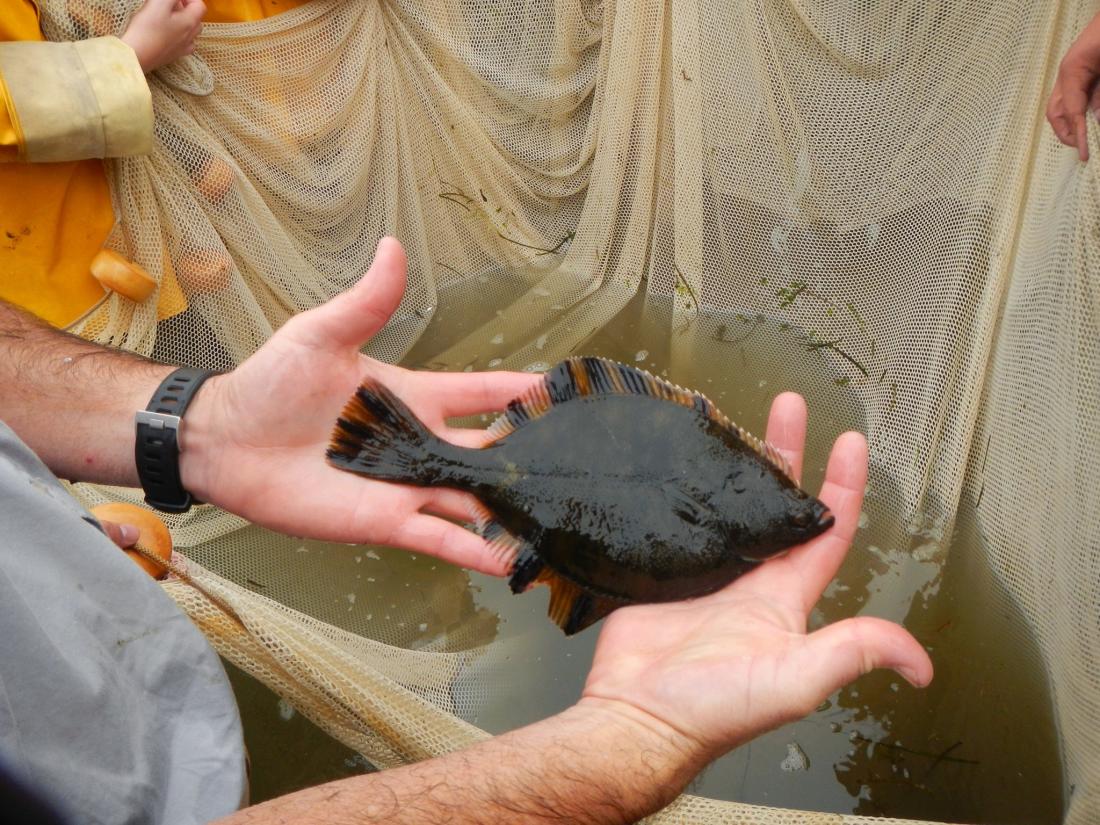In this vivid photograph, a man is holding a small, dark green-black fish with a slightly slimy appearance, cradled in his palm and a half. The fish, resembling a bottom feeder and about the size of the man's hand, has a flat, fat oval shape. Its face, turned towards the camera, displays two small eyes and a triangular mouth slightly ajar. The fish's fins, adorned with striking vertical brown and black stripes, extend from its top and bottom. 

Behind the man, a standard fishing net with orange weights is held aloft by multiple hands, including one that appears to belong to a child. The net is filled with murky water and some entrapped greenery, indicative of the dirty freshwater it came from. A person clad in a yellow raincoat is visible at the top left corner, contributing to the scene. 

The photograph captures a sunny day with notable contrast and vivid coloration, making the details of the shiny, wet fish and the surrounding environment pop. Additionally, a black wristwatch is noticeable on the man's left arm, subtly emphasizing his grip on the caught fish.